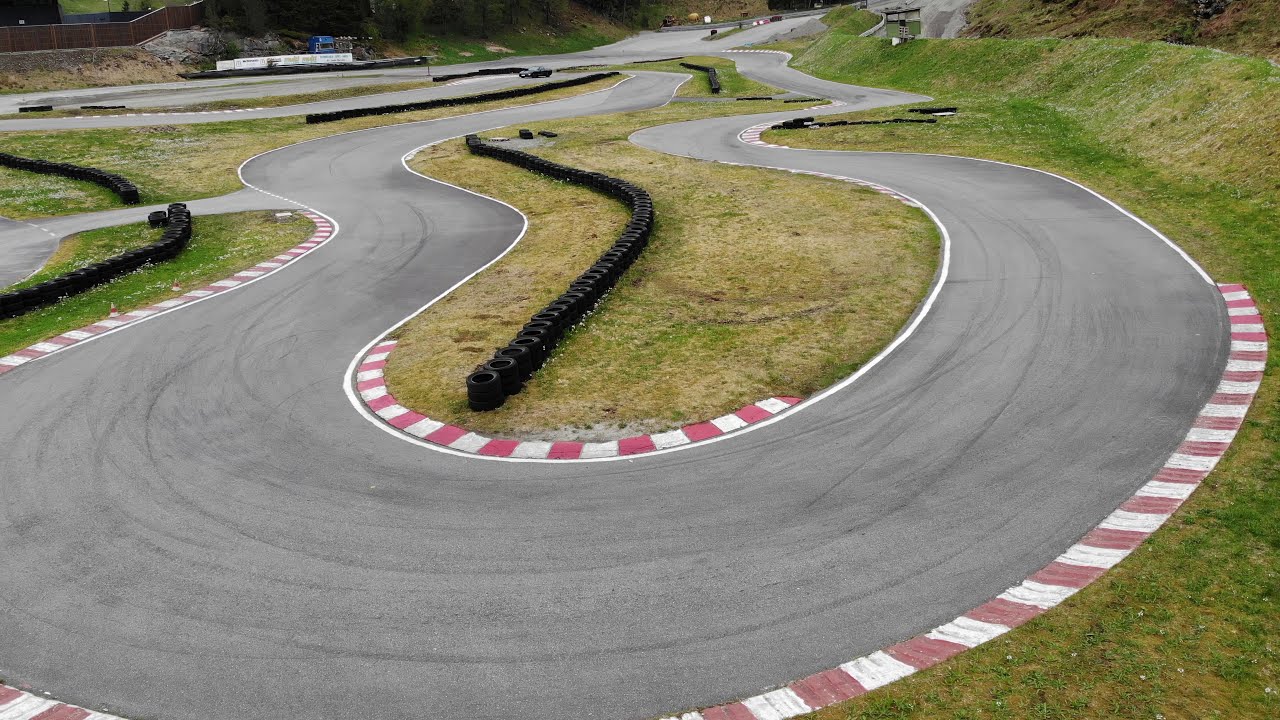The image depicts an intricate go-kart racetrack characterized by its serpentine layout starting from the top center and winding through numerous tight turns, resembling a snake as it descends. The track makes a series of turns to the right and left, descends to the bottom, makes a sweeping U-turn towards the bottom left, and then ascends again with more twists and turns before reaching a main straight in the back. The gray asphalt of the track is visibly scratched with black skid marks, indicative of frequent high-speed maneuvers. Red and white patchwork barriers line the track's edges, providing clear visual demarcation against the adjacent grass, which is a blend of green and yellow shades. Safety barriers consisting of rows of black tires are strategically placed at various points around the track. 

In the distance, a highway with a few vehicles can be seen, adding depth to the scene. On the right, the track ascends a gentle grassy slope before encountering a steeper mountain bank. The upper left corner features a wooden barrier accompanied by a dirt bank, enhancing the rustic outdoor environment. The track's expansive and challenging design, coupled with its safety features and outdoor setting, suggests it's suitable for experienced drivers looking for an adrenaline-filled experience.